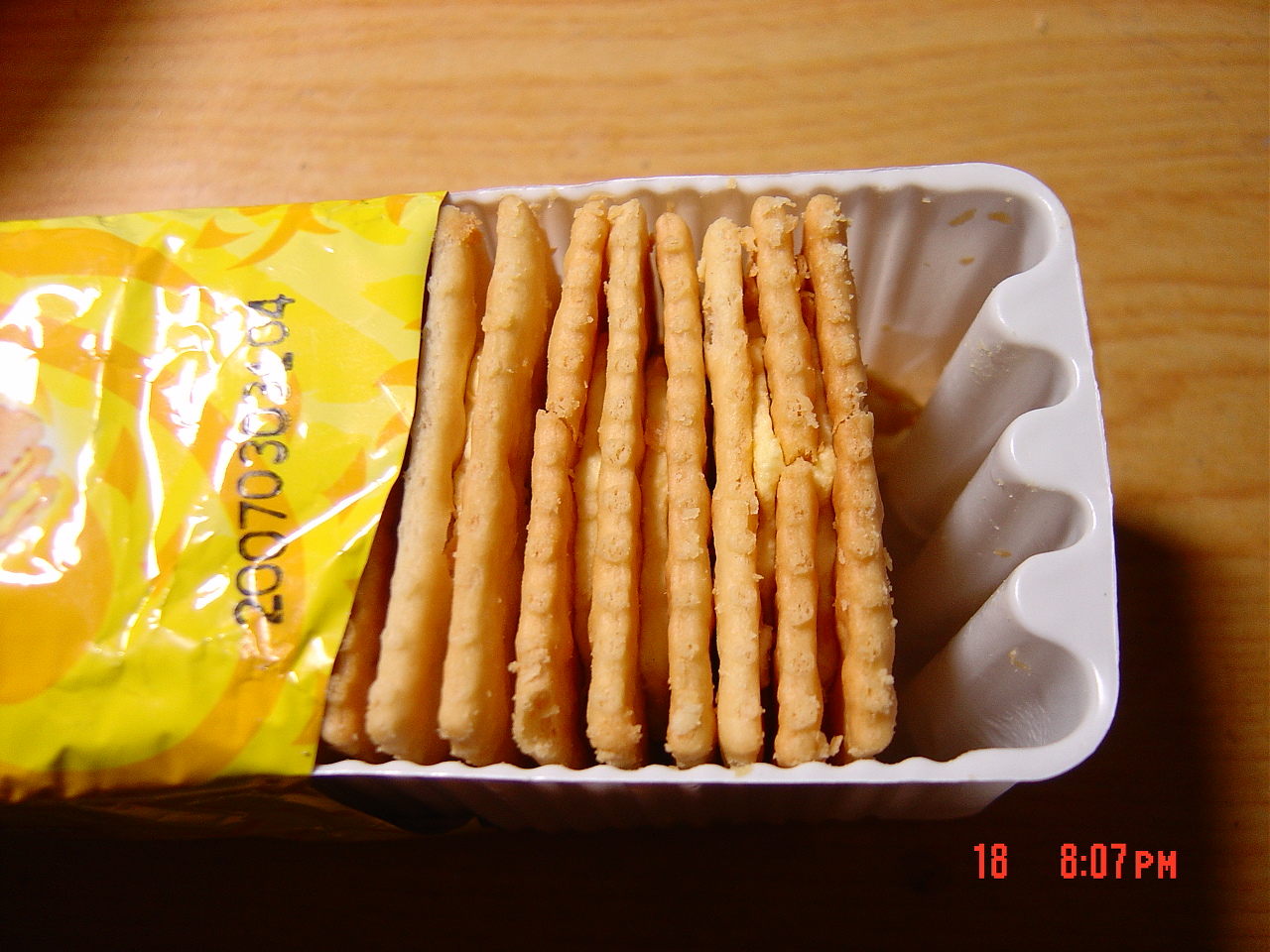This image features a package of snack sandwiches composed of cheese and crackers. The sandwiches are arranged as triple-decker units, each consisting of three crackers with two layers of cheese between them. The plastic package is predominantly yellow with an orange design, partially obscured by glare, making the pattern indiscernible. The edge of the package shows crumbs clinging to the sides. A number, "2007030" and possibly "34 04" can be seen printed on the package amidst the glare. The sandwiches are housed in a white plastic tray, pulled partially out from its plastic wrapper, revealing some cracked units. The scene is set on a light brown wooden table. In the lower right corner of the image, the time "18:07 p.m." is displayed in red numbers.